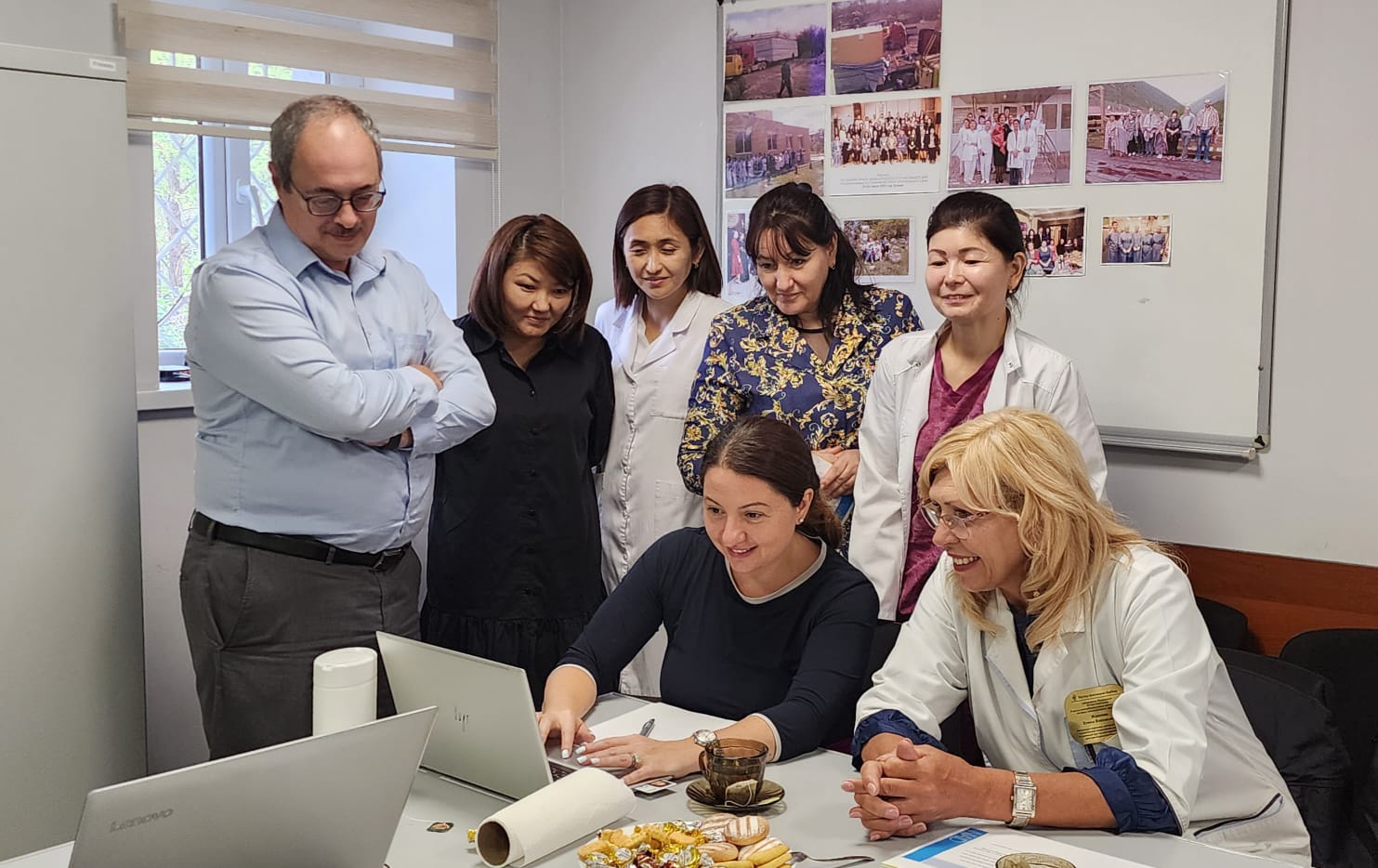In the image, a group of seven individuals is gathered around a desk, focused intently on a computer screen being worked on by a middle-aged woman with brown hair, wearing a dark blue long-sleeve shirt. Her hands are on the HP laptop, with two people seated beside her and five standing behind. The scene appears to be in an office setting, indicated by the light gray walls, pictures, and a bulletin board in the background. To the left, an open window lets in sunlight.

From left to right, the standing individuals include:
1. An older white male in a light blue office shirt and gray dress pants.
2. A woman in a black jacket.
3. A woman wearing a white jacket and pink undershirt.
4. A woman in a black and gold dress.
5. An older woman with gray hair, a white jacket, and a watch on her arm.

Seated next to the woman at the computer are:
1. A woman wearing a floral blue shirt.
2. A middle-aged Latina woman in a lab coat.

A second computer sits idle at the bottom left of the table, next to a cup of tea and a plate filled with cookies. Everyone except for one woman, who seems less animated but still engaged, is smiling and appears deeply engrossed in whatever is displayed on the laptop screen, which could be anything from a TikTok video to a work project.